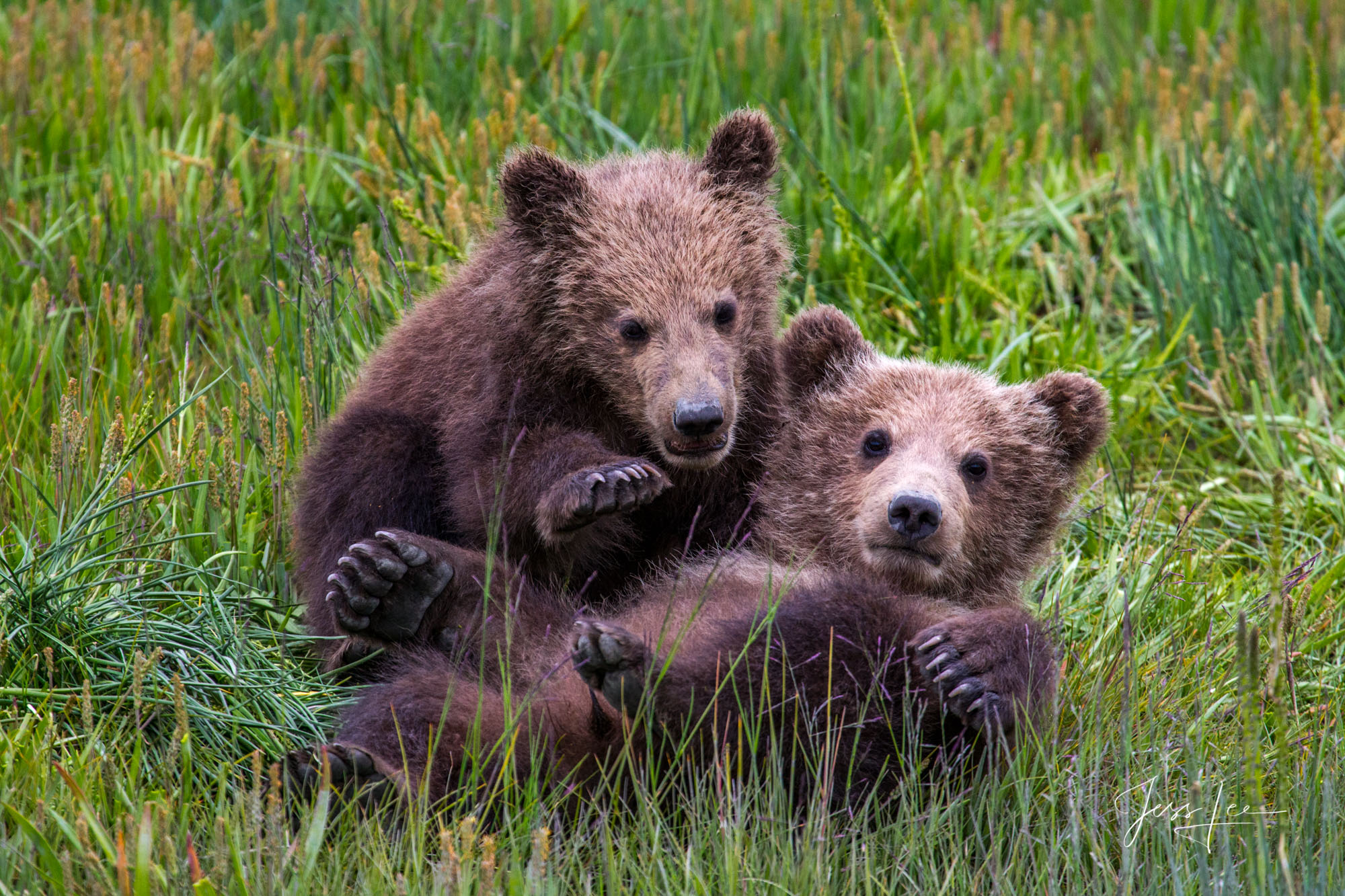This image captures two small, brown bears playfully interacting in tall, un-mowed grass of varying shades of green and hints of orange and brown. The scene is set during the daytime. Centrally framed, one bear lies on its back with its head slightly tilted to the right and its limbs, including its sharp claws, raised in the air, directly facing the camera with an inquisitive look. Next to it, the second bear is partially seated on its hind legs, reaching its front paw towards the belly of the bear on its back. Both bears have lighter-colored fur around their noses and foreheads, with the bear lying on its back having a slightly lighter tummy and darker back. The composition captures the intimate and playful nature of these young bears amidst the dense grass, which obscures any background elements, focusing the viewer's attention on their interaction.